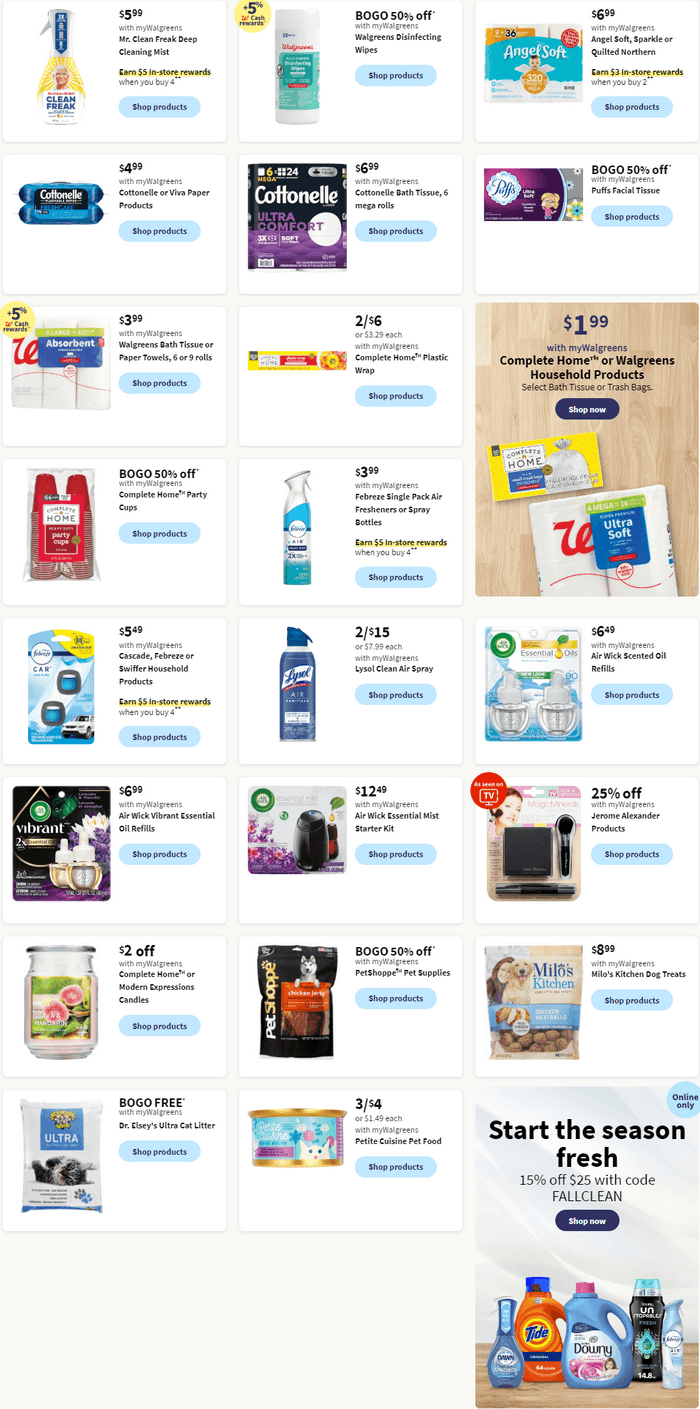This image is a detailed coupon page, likely sourced from Walgreens, as indicated by a prominent red "W" logo. The layout features multiple sections showcasing various cleaning products and household items. 

In the upper portion, there is a brown-highlighted section displaying paper towels. Adjacent to this, slightly obscured, is another segment with the Walgreens logo partially visible. Moving towards the lower middle of the page, a third image from the left depicts toilet paper prominently displayed with sale information, again featuring the red "W" signifying Walgreens.

The page is densely packed with product images, organized into three columns across and approximately ten rows down, ensuring a comprehensive visual presentation of the available deals. At the very bottom, a large box stands out with a seasonal promotion. It reads "Start the Season Fresh" and offers a 15% discount on $25 purchases using a specific code, encouraging online shopping. Five cleaning products in a variety of colors—orange, blue, black, and light blue—are pictured next to this promotional message.